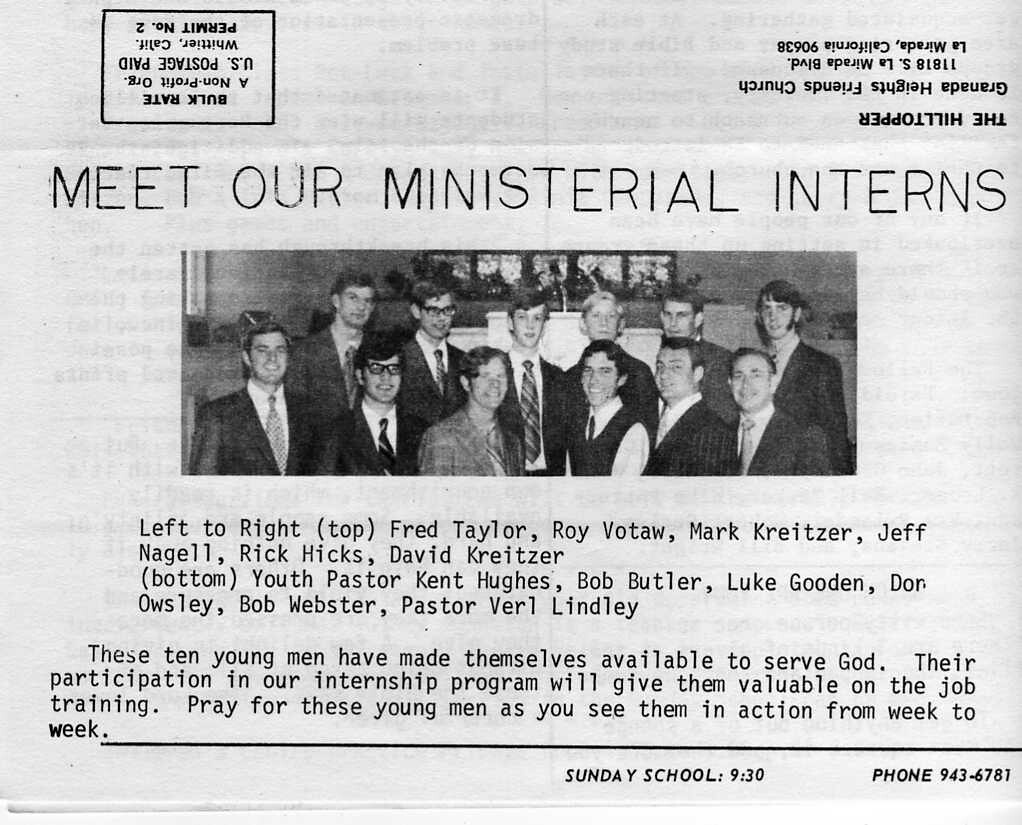The image appears to be a scan of a mailed church newsletter from the Granada Heights Friends Church, located at 11818 South La Mirada Boulevard, La Mirada, California, 90638. The title at the top of the page reads "The Hilltopper." This folded-over page displays an upside-down bulk postage stamp in the upper left corner. The main segment of the scan prominently features the heading "Meet Our Ministerial Interns" in thin, capitalized letters. Beneath this heading is a black-and-white photograph of twelve young men, all dressed in suits and ties, with one in the foreground wearing a vest and tie. The arrangement of names listed identifies the twelve individuals from left to right; the top row includes Fred Taylor, Roy Votaw, Mark Kreitzer, Jeff Miguel, Rick Hicks, and David Kreitzer. The bottom row includes Youth Pastor Kent Hughes, Bob Butler, Luke Gooden, Don Owsley, Bob Webster, and Pastor Verl Lindley, who are standing in front of a stained glass window with flower beds. A paragraph accompanying the photograph reads: "These ten young men have made themselves available to serve God. Their participation in our internship program will give them valuable on-the-job training. Pray for these young men as you see them in action from week to week." At the very bottom of the page is a line separating the paragraph from additional information, which states "Sunday School 9:30," followed by the phone number "943-6781" in the bottom right corner.